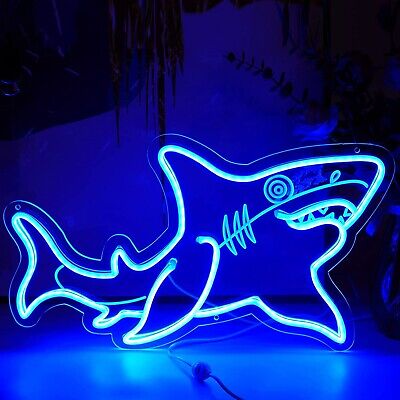The image depicts a vibrant blue neon sign of a stylized, almost cartoonish depiction of a shark, facing the viewer's left. The shark is crafted with elaborate details: three lines run down its side, and its eye is crafted from three concentric circles. A single nostril is visible above its slightly open mouth, revealing six teeth. The full body of the shark is on display, including its tail, fins, and what might be referred to as arms. The neon sign appears to be made from neon tubing affixed to a flat sheet of plexiglass or similar material. The background is dimly lit with hints of dark blue hues, possibly suggesting plants and a shelf in a domestic setting. The sign is likely positioned on a light blue table, with the reflection of the neon light casting an ethereal glow upon it.